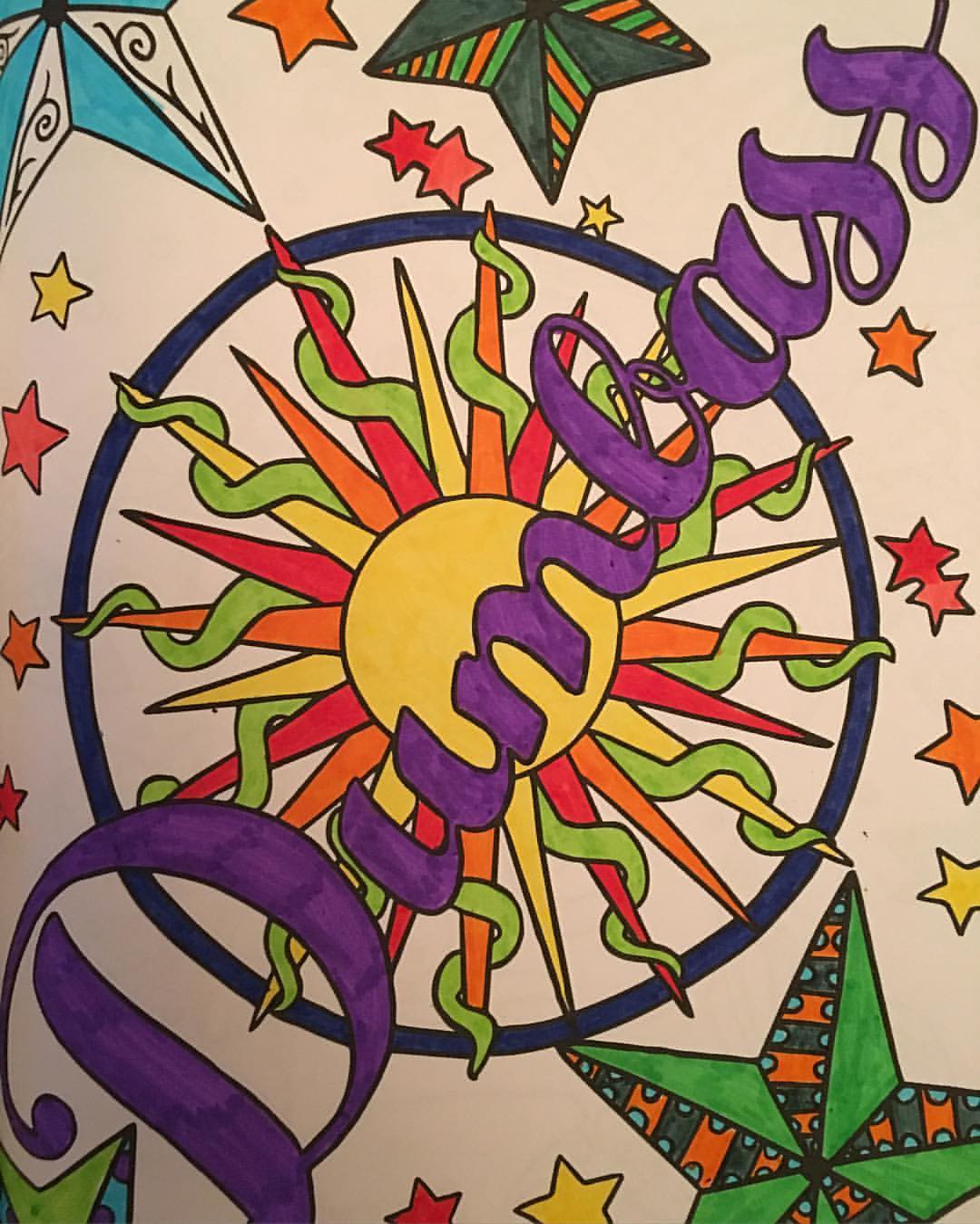This is a colorful poster on a white background, featuring a prominently written word "dumbass" in thick, purple cursive lettering across the center. The primary visual element behind the text is a bright yellow sun with multi-colored rays extending outward. The rays are red, orange, and yellow, and around some of them are green, tentacle-like tendrils. The sun is encased in a dark blue circle. Beyond this circle are numerous small stars in shades of yellow, red, and orange. There are also larger, more detailed stars with varied colors and patterns: a striped green and orange star is at the bottom right, a blue and white star is at the top left, and another green and orange star above. The poster has a vibrant and whimsical aesthetic, combining cosmic elements with bold, playful design.